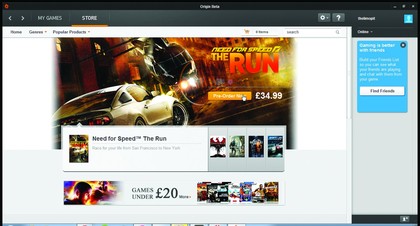A detailed screenshot of a computer screen primarily features a gaming platform interface overlaying an indiscernible background. The visible window displays a navigation bar at the top in a charcoal gray color, with tabs labeled "My Games" in a lighter charcoal gray and "Store" highlighted in white, indicating it's the selected section. To the right of these tabs, a magnifying glass icon allows for search functionality, followed by a question mark for help or support.

Beneath this, a white bar provides navigation links including "Home," "Games," and "Popular Products," while a search bar is positioned at the far right. Dominating the central part of the interface is a prominent promotional graphic featuring a Ford Mustang spinning out in front of a helicopter, advertising the game "Need for Speed: The Run" with an option to click on a gold button for purchase details. The game is priced at £34.99 and offers various versions. 

Below this main feature, there's a section highlighting budget-friendly options with a banner "Games for under £20," showcasing multiple game thumbnails. This interface setup clearly aims to attract gamers searching for new titles and deals.